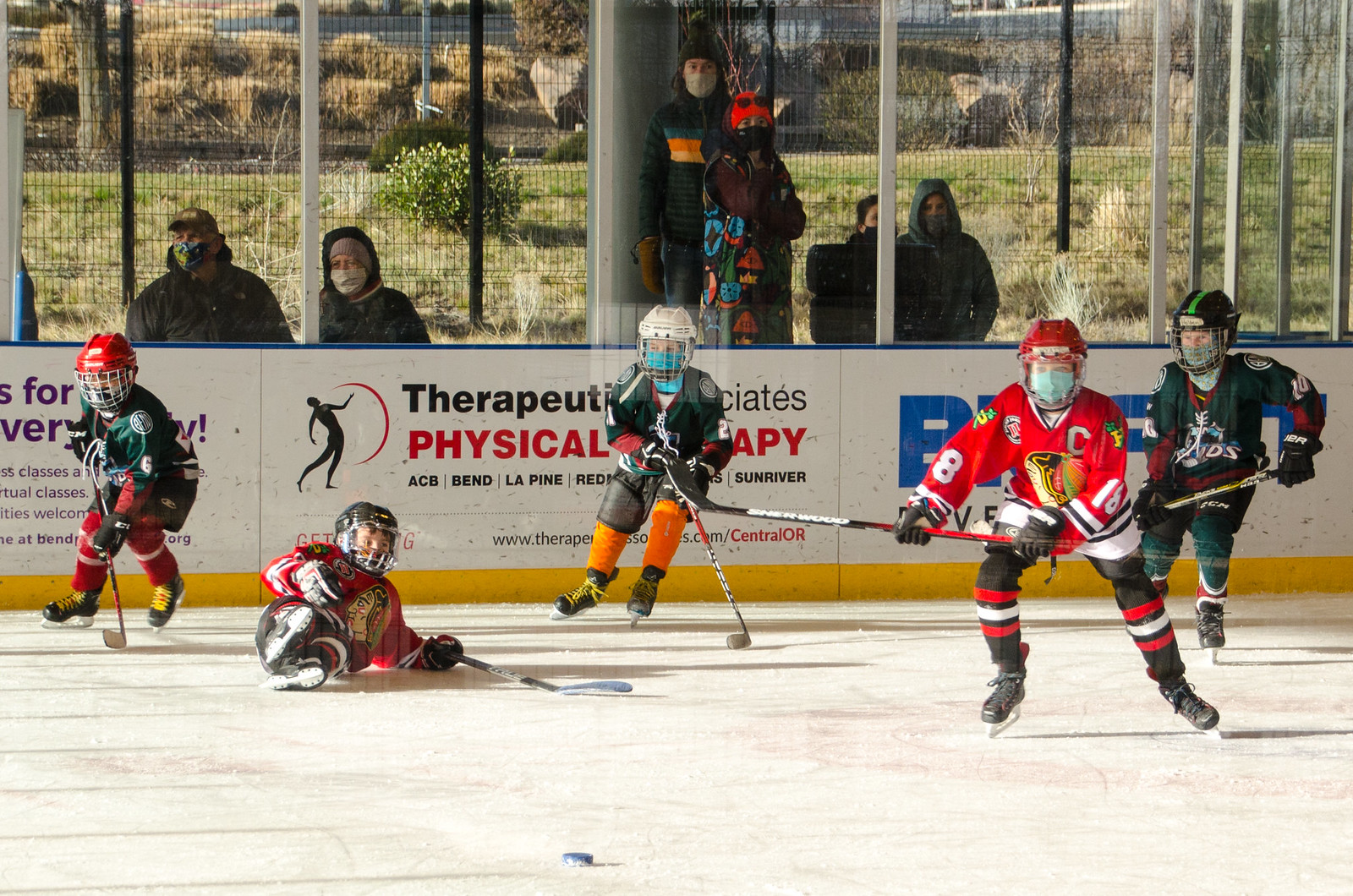The photograph, seemingly taken by a professional specializing in youth sports, showcases a youth ice hockey game. The scene unfolds on an indoor rink that seems to blend into an outdoor setting, likely in a place with a warmer climate like Arizona. On the ice, five children are engaged in the game, dressed in full protective gear, with varied uniforms in colors predominantly red, black, green, and white. One player has fallen, while the puck is visible nearby. 

The rink is encased by a wall displaying advertisements, including one for "Therapeutics Physical Therapy." Behind this barrier, three couples, clad in winter attire including jackets, hats, and hygiene masks, are intently watching the game. Through the glass that separates the spectators from the rink, an incline of greenery with both lush and dried plants, and a building in the far distance, can be seen, adding to the blend of indoor and outdoor elements of the setting.